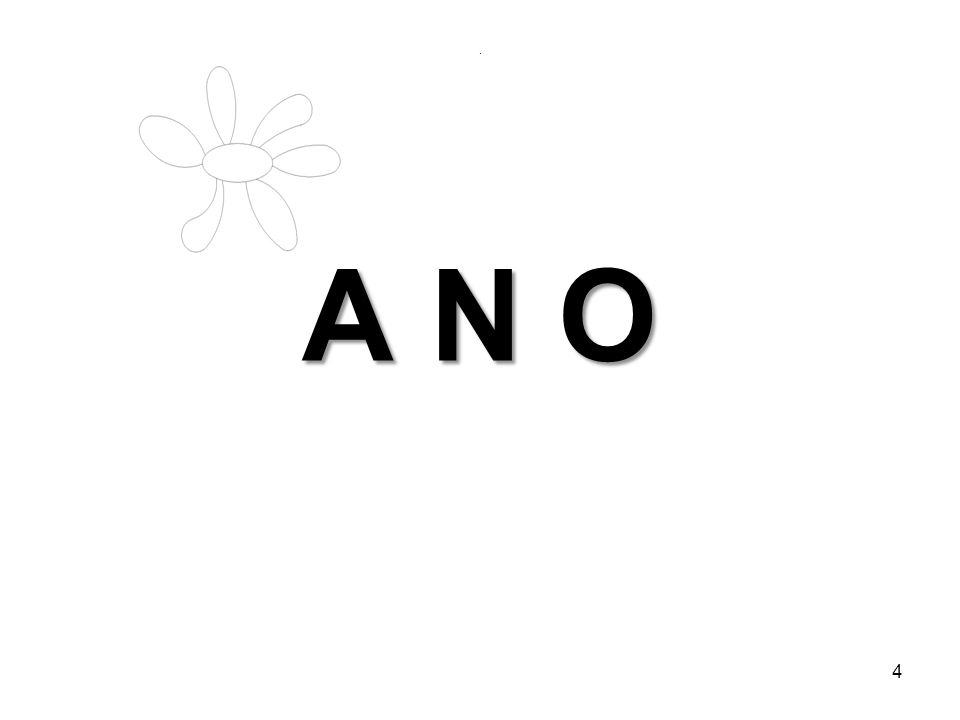The image displays a minimalistic design, featuring a stark white background with a few distinct elements: an illustration and text. In the upper left corner, there is a lightly drawn, digitally created flower comprised of an assortment of petals with varied shapes—some ovals, some elongated, and others slightly curvier—arranged around a central oblong shape and notably lacking a stem. Centered in the image is the bold black text "A-N-O" in capital letters, spaced distinctly apart. In the bottom right corner, the page number "4" is displayed in black. The combination of these elements, along with their arrangement, suggests that this image may be a page excerpt from a book. The color palette is strictly monochromatic, utilizing only shades of gray and black against a white background.